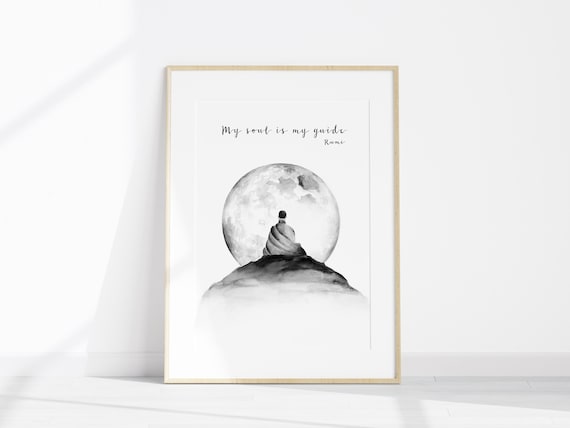This image captures a rectangular piece of artwork positioned against a light gray, almost white wall, with its bottom resting on a flat surface that could be a shelf, table, or countertop. The artwork is vertical and framed in light brown or tan wood, with a white border surrounding a black-and-white scene. In the center of the artwork, a man is depicted sitting on a hillside, cloaked in robes, with his back to the viewer. He gazes at a large, detailed moon that dominates the upper portion of the image, creating a halo effect around him. Above this serene scene, the text "My soul is my guide" is prominently displayed in black, followed by the name "Rumi" underneath. The overall aesthetic suggests a watercolor style, emphasizing the contemplative mood of the piece.